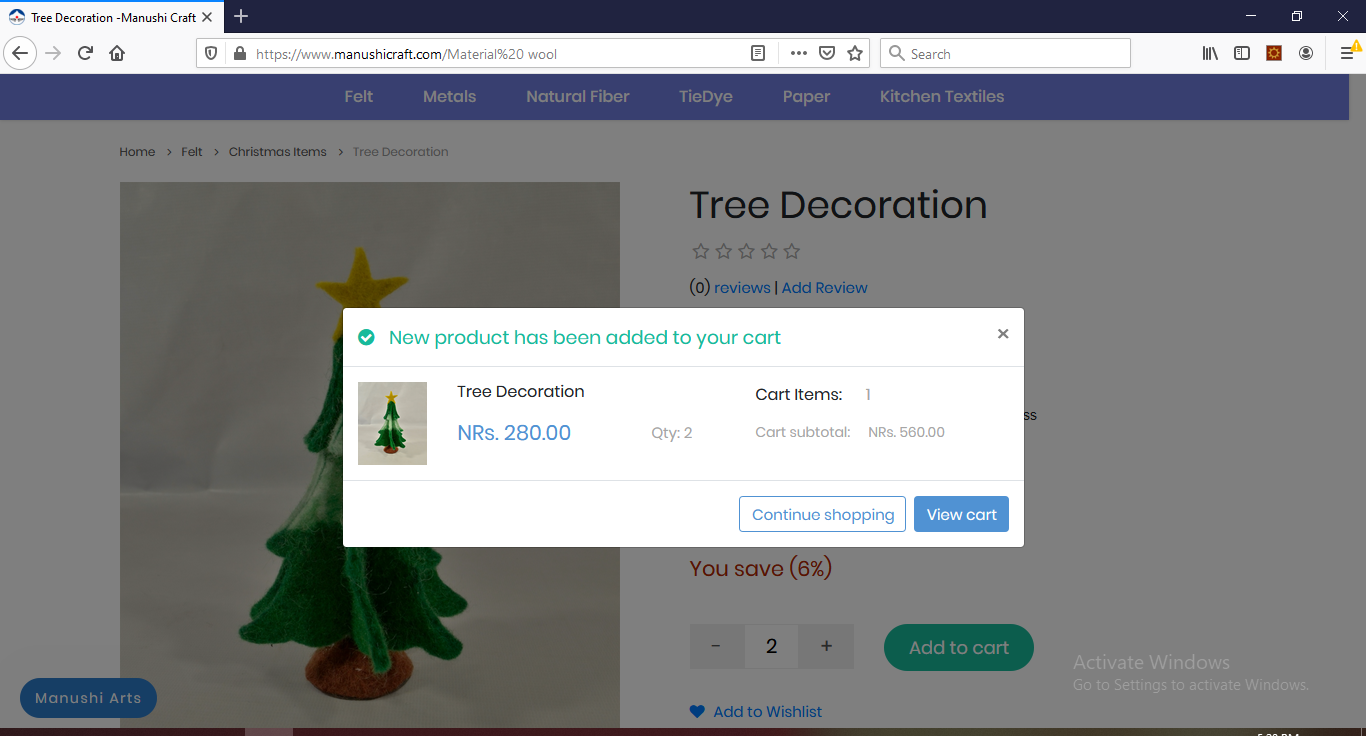**Screenshot Description of ManushiCraft Website**

At the top of the webpage, there is a dark navy blue navigation bar with the title "TreeDecoration - ManushiCraft" prominently displayed on the left. This bar includes several standard web navigation elements: a back arrow, a circle, a grayed-out right arrow, a refresh button, a home button, a shield icon, a lock icon, and the URL "https://www.manushicraft.com/material%20wool". Adjacent to the URL are icons for a page, a vertical line, three dots, a shield with a check mark, a star, and a search box.

Below the navigation bar is a white notification box informing the user of a new product added to their cart. This notification features a green circle with a white checkmark and the text "New product has been added to your cart." There is an "X" on the right-hand side to close this message.

The notification box contains a small image of a tree decoration consisting of a small tree on a red base with a yellow star at the top. The caption beneath this image reads "Tree Decoration" with the price "NRS. 280.00" in blue. Details about the quantity "Quantity: 2", "Cart items: 1", and "Cart subtotal: NRS. 560.00" are presented, followed by buttons to "Continue Shopping" and "View Cart".

Further down, the main content of the grayed-out page is still visible. A blue bar at the top lists product categories like "Felt", "Metals", "Natural Fiber", "Tie-Dye", "Paper", and "Kitchen Textiles". Below this is a breadcrumb trail indicating the navigation path: "Home > Felt > Christmas items > Tree Decoration". 

In large black text, the product name "Tree Decoration" is displayed, accompanied by five empty white stars indicating the absence of product reviews, and an "Add Review" option. The same image of the tree decoration appears enlarged beneath this section.

Product details include a red message stating "You saved 6%", a quantity selector displaying the number "2" between plus and minus buttons, a green "Add to Cart" button, and a blue heart icon for adding the product to the wishlist. To the right of the "Add to Cart" button, a message prompts the user to "Activate Windows" and visit the settings to do so.

Finally, at the bottom left corner of the page, there is a blue oval with the text "Manushi Arts".